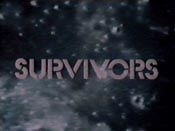The image appears to be computer-generated and showcases a night sky or a deep space scene as the background. The backdrop is a dark expanse filled with an array of white spots and grayish-white swirling patches, reminiscent of stars and nebulas typically observed in space photography. The outer edges of the image are especially dark, enhancing the cosmic setting.

In the foreground, the word "SURVIVORS" is prominently displayed in all capital letters, rendered in a light gray hue. Each letter exhibits an intriguing pattern, with most letters featuring a distinct division that slices through them. Specifically, the "S" is split horizontally in the center, the "U" is divided at the bottom, and the "R" is segmented in two places—between the curved and the straight parts, as well as at the leg. This halving effect continues for all the letters except the "I," which remains solid and undivided, standing as a singular contrast to the fractured aesthetic of the other characters.